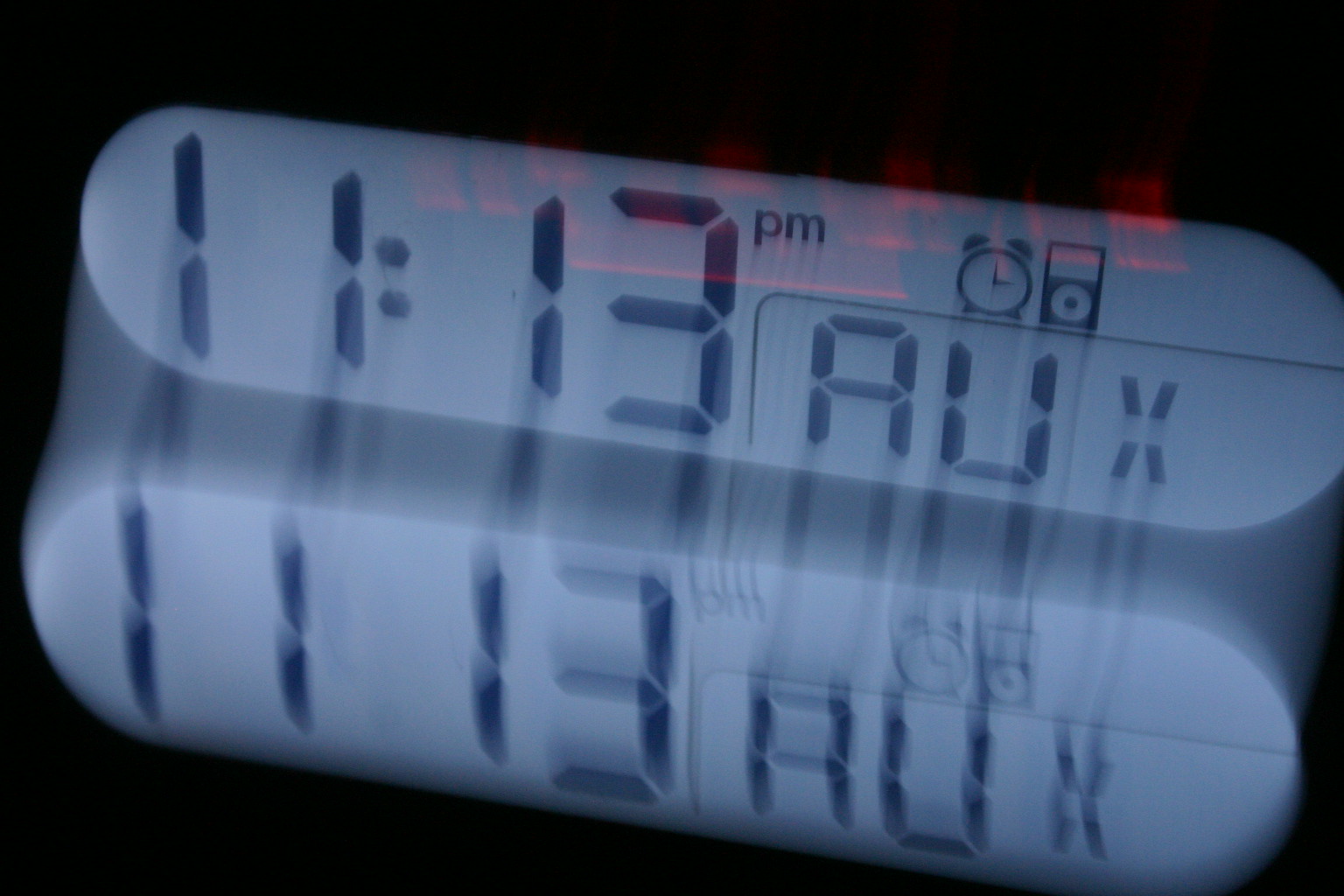The image depicts a blurry digital alarm clock face set against a completely black background. The clock display shows the time as "11:13," with the digits appearing in either navy blue or black on a light blue or dark white backdrop. On the right side of the display, there is a half-square with rounded edges labeled "AUX," accompanied by symbols representing a clock and an iPod. Notably, the entire image is doubled and reflected below the original display, creating a mirrored, blurred effect where the same elements, including the time, "AUX" label, and symbols, are repeated directly underneath the initial display. The overall effect is a disorienting, doubled vision of the alarm clock face.